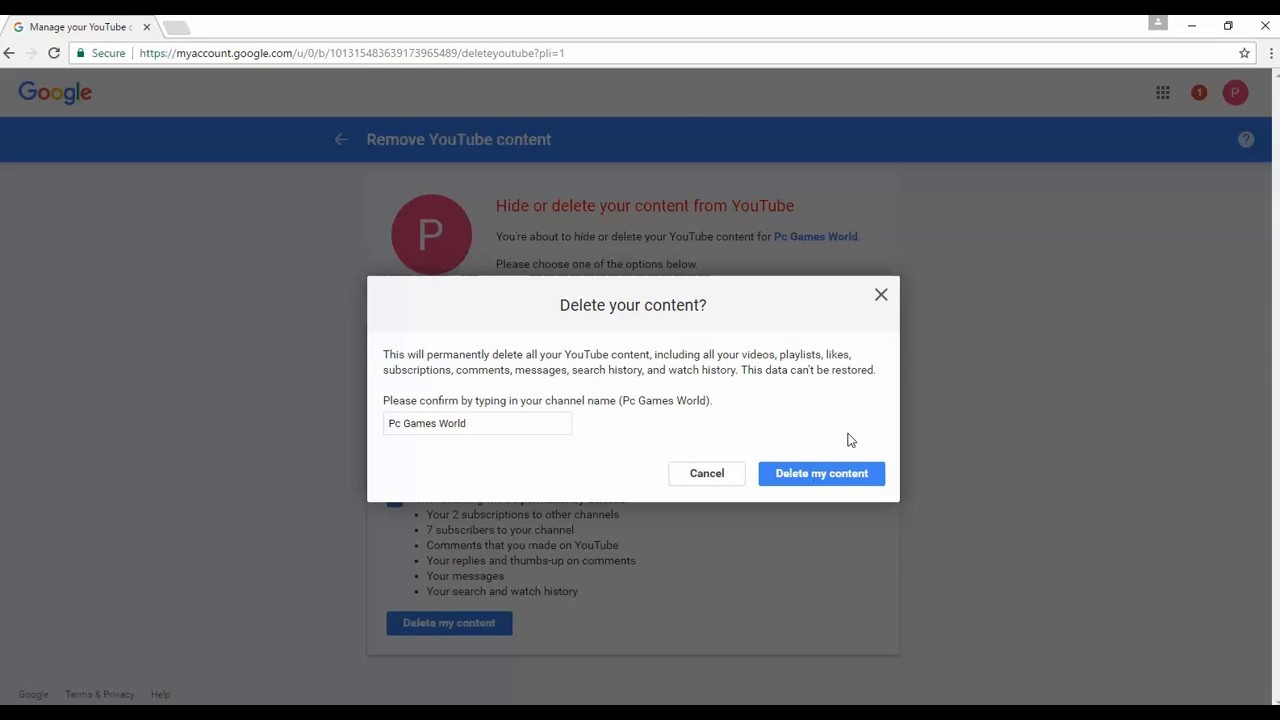The image is a screen capture of an older version of the Google Chrome web browser, showing a user logged into their Google account, specifically within the main settings area focusing on YouTube account management. Prominently displayed in the center of the browser window is a dialogue box titled "Delete your content," which warns the user about the implications of their action. The box offers two buttons: "Cancel" and "Delete my content," giving the user a final choice to either proceed with or abort the deletion process. The background of the screen is dimmed, highlighting the foreground dialogue box to emphasize the user's decision. 

In the dimmed background, part of the interface can still be discerned. At the top, the Google logo is visible, accompanied by a blue navigation bar just beneath it. The label "Remove YouTube content" is displayed within this bar. Also noticeable is the user's icon—a red circle featuring the letter "P." Next to this icon, the text "Hide or delete your content from YouTube" is partially readable, followed by additional grayed-out text. The overall scene clearly depicts a critical moment where the user is about to decide whether to permanently remove their YouTube content.